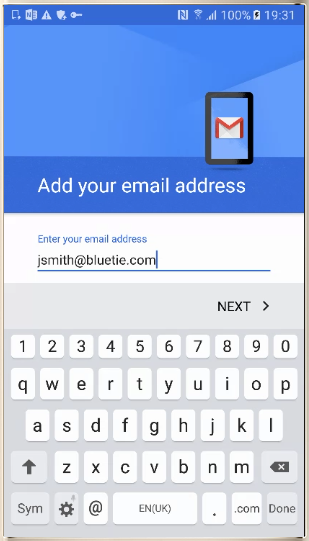This is a detailed descriptive caption of a mobile phone screenshot:

The screenshot displays a mobile phone interface at 19:31, with full Wi-Fi and signal strength, and a 100% battery level, indicated at the top by a blue bar containing various icons: a key, a shield, and a warning triangle with an exclamation mark. Directly below this bar is a blue square featuring a smartphone icon with an envelope. Beneath the blue square, a darker blue bar contains the white text "Add your email address." Below this bar, a white rectangle prompts the user in blue text to "Enter your email address." The user has started inputting their email address, "bluetie.com," using the gray-background mobile keyboard visible at the bottom. The keyboard features characters in a standard layout, with the keys marked "Next" at the top and a sequence of alphanumeric characters, including the numbers 1 through 0 and the letters Q through M, along with an up arrow.